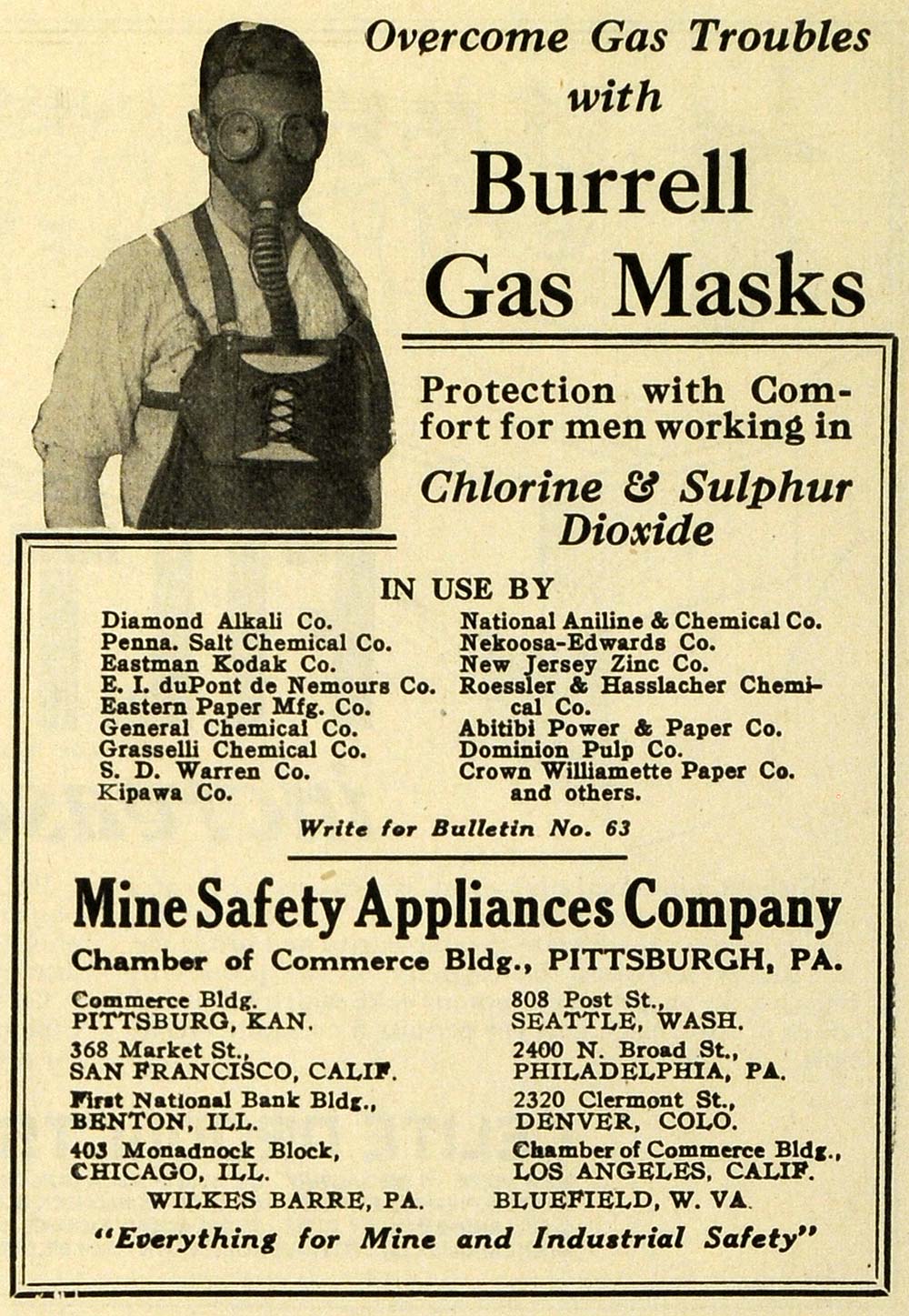This vintage poster serves as an advertisement for Borel gas masks, prominently featuring the slogan "Overcome gas troubles with Borel gas masks." In the upper left corner stands a man wearing a collared button-up shirt and an apron, modeling an old-fashioned gas mask. The background is beige with black text, suggesting it may have been printed in a newspaper. Below the main slogan, the poster highlights "Protection with comfort for men working in chlorine and sulfur dioxide," and lists the companies that use these masks, such as General Chemical, Diamond Alkali, Kipawa Company, and National Aniline and Chemical Company. At the bottom, the advertisement notes, "Write for bulletin number 63, Mine Safety Appliance Company, Chamber of Commerce Building, Pittsburgh, Pennsylvania," and concludes with the line "Everything for mine and industrial safety."